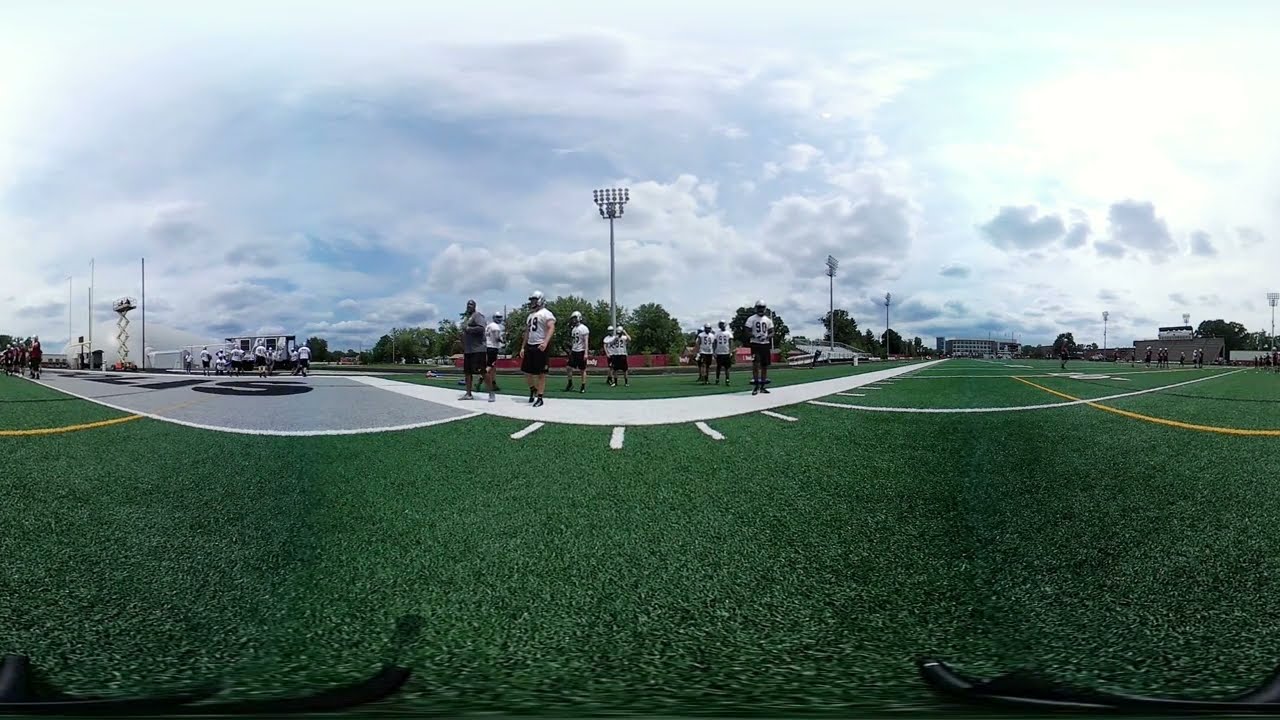The image captures a football field during a cloudy day, taken from almost ground level. The green grass of the field is prominently featured, marked by a long white line with several smaller lines intersecting at regular intervals of about two feet. Towards the center, there is a large patch of grass painted white with visible black letters "L-I-S." In the foreground, seven football players in white helmets, white jerseys, and black shorts stand in between plays, presumably receiving instructions from a coach in a gray sweatshirt. Surrounding this central scene, additional football players are visible in the background, lined up as if in the middle of a game or practice drill. On the right side, there are towering field lights that are turned off, as well as a scissor lift extended in a fully upright position with more players gathered near it. The left side features a team logo with some distorted text, hinting at the use of a 360-degree camera for capturing this expansive field. The backdrop showcases large, cloudy skies with intermittent breaks of blue, adding to the dynamic atmosphere of the scene.